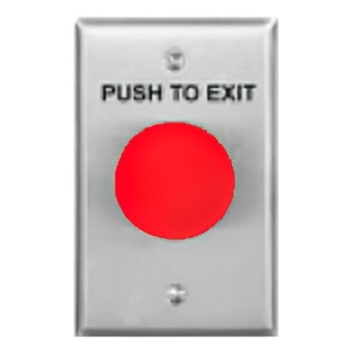The image depicts a centrally positioned, metallic rectangular faceplate with a beveled edge, similar to a light switch or outlet cover. It is affixed to a completely white background using screws located at the top and bottom center of the faceplate. Dominating the center of the faceplate is a prominent red button. Above this button, framed by the metallic surface, are the bold black words "PUSH TO EXIT." The faceplate, a silver-gray color, appears to be intended for indoor use, possibly as an emergency escape or door release button in a commercial or business setting.